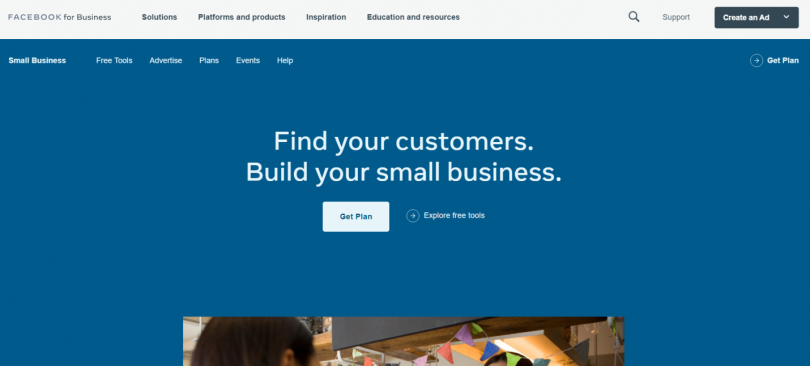This panoramic image appears to be a section from a business-oriented website, specifically for Facebook. At the very top, a long gray navigation bar houses multiple menu items for users to click on. On the upper left, bold black text reads "FACEBOOK FOR BUSINESS," and from left to right, additional clickable black text options are visible: "Solutions," "Platforms and Products," "Inspiration," "Education and Resources." 

To the right of this menu, a search icon depicted as a black magnifying glass is complemented by the word "Support" in gray lettering. In the upper right corner, there is a deep blue text box with white lettering that reads "Create an Ad," accompanied by a downward-facing gray arrow, indicating further options can be accessed by clicking.

The larger section of the image features a blue background with various elements. In the upper left corner of this blue section, white text lists additional navigable categories: "Small Business," "Free Tools," "Advertise," "Plans," "Events," and "Help." On the far right, a prominent white circle with a blue interior contains a right-facing white arrow, next to the white text "Get Plan."

Centrally located within the image, large white text delivers the message: "Find your customers, build your small business." Below this, a clickable white box with blue text reads "Get Plan," flanked by a similar white-rimmed circle with a blue interior and a white right-facing arrow, next to which the text "Explore Free Tools" is visible.

At the very bottom center of the image, a partially visible photograph captures only the top portion of an individual’s head with brown hair. The background includes some indistinct pendants and ceiling lights, but the rest of the photograph is cut off, making it hard to discern further details or context.